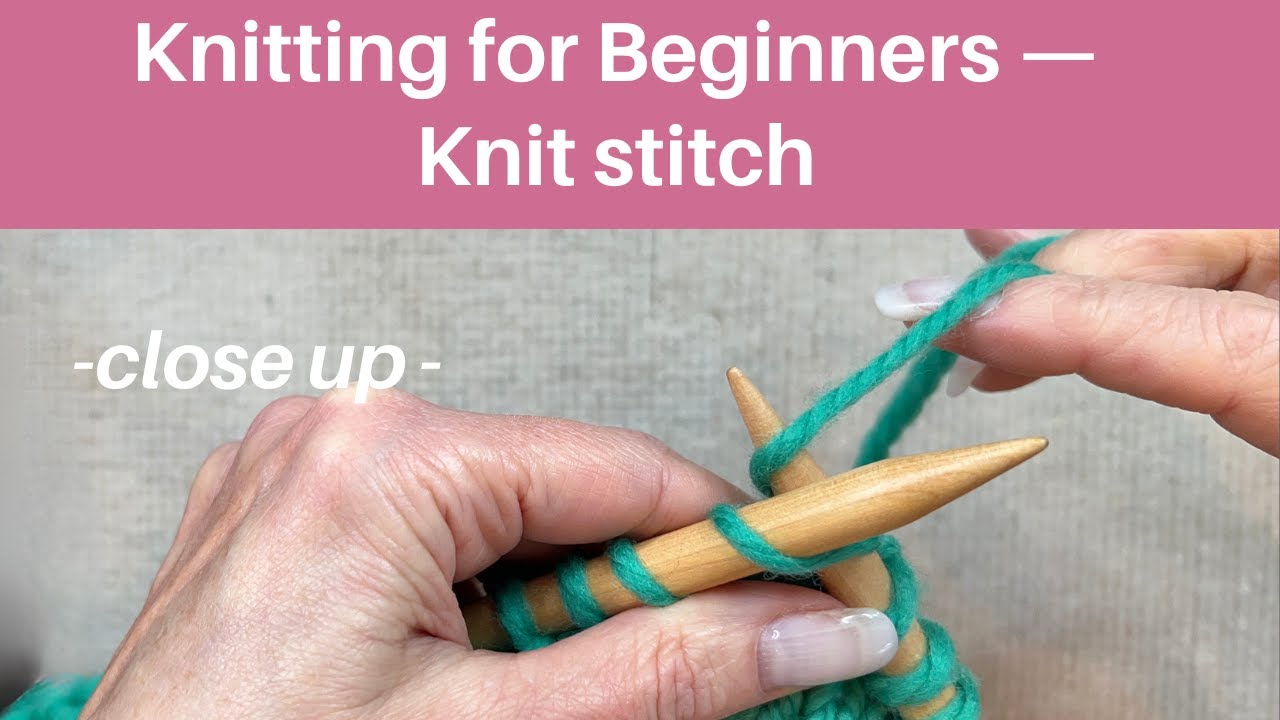The image is a horizontally rectangular, full-color photograph with a staged, indoor setup using artificial light. A dark pink banner runs across the top, prominently displaying the text "Knitting for Beginners - Knit Stitch" in bold, white lettering. Below the banner, the focal point of the photograph is the close-up of two well-manicured Caucasian female hands engaged in knitting. The nails are long and finished with a clear polish. One hand holds a wooden knitting needle in the left, while the other hand manipulates another needle and a piece of blue-green yarn, demonstrating the initial stages of the knitting process, specifically casting on stitches. Some stitches are already visible on the right-hand needle. The background is a grayish material that contrasts with the hands and the yarn. To the right, the word "Close-up" is annotated, ensuring viewers focus on the meticulous knitting technique displayed. This advertisement likely targets beginners interested in learning how to knit.